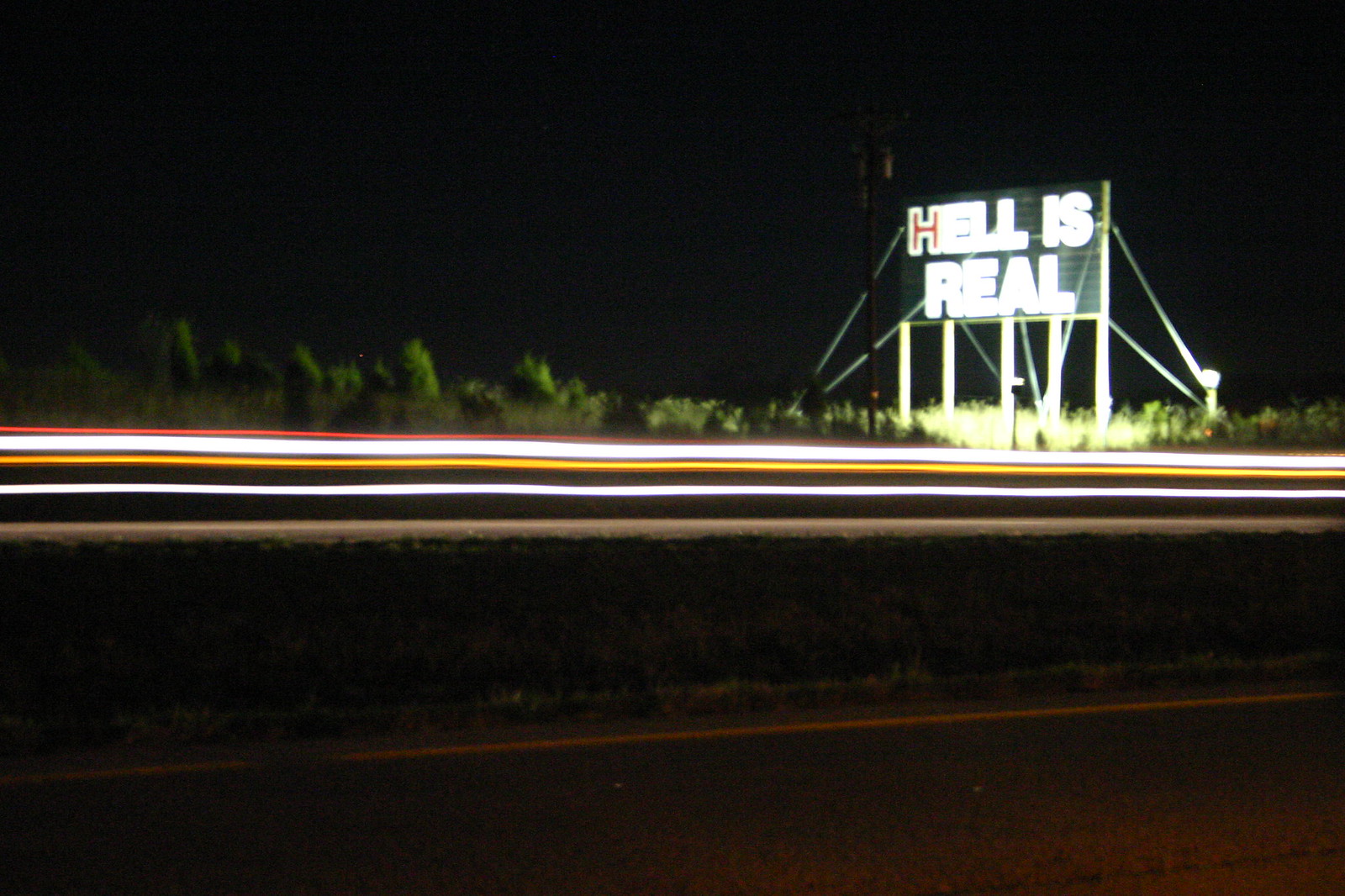This nighttime photograph captures a foreboding scene along a dark, deserted road. Dominating the frame is a large billboard mounted on sturdy wooden posts. The billboard's background is black, creating a stark contrast with the large white letters that spell out "HELL IS REAL," except for the ominously red letter "H" that begins the phrase. The sign is illuminated by an overhead spotlight, casting an eerie glow.

In the foreground, streaks of orange, white, and amber lights blur together, suggesting the recent passage of vehicles, adding a sense of motion and urgency to the still night. To the right of the billboard stands an indistinct electrical pole, its details obscured by the darkness. Surrounding the road, sparse brush and vegetation are barely visible in the low light, contributing to the desolate and haunting atmosphere of the scene.